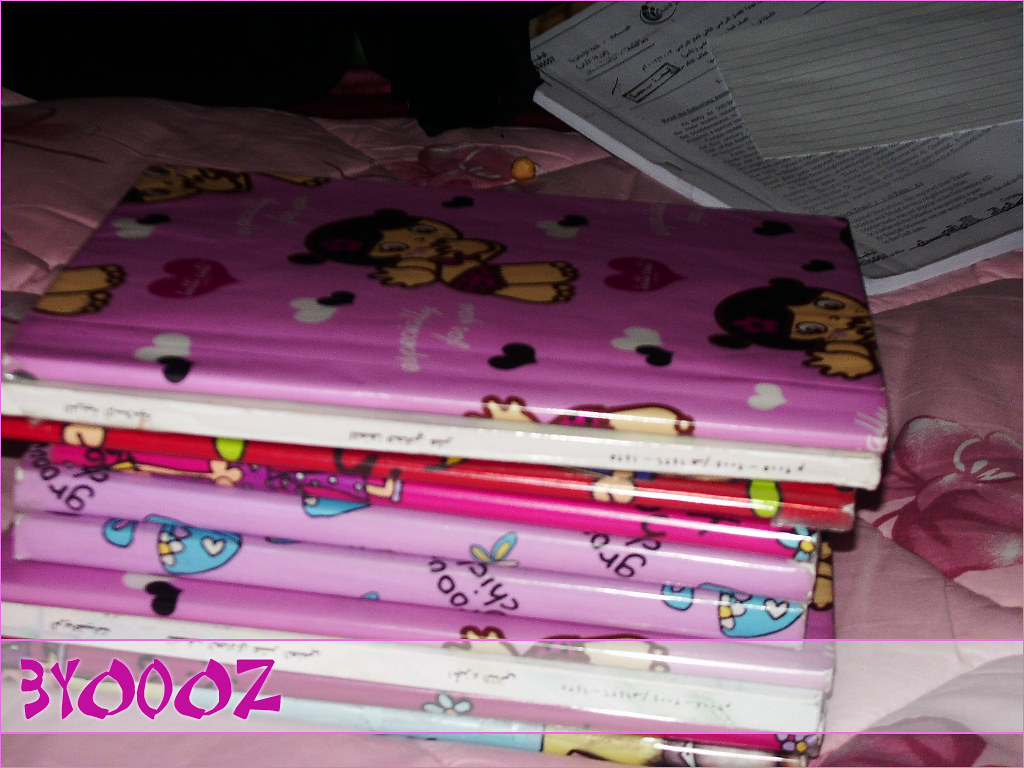The image features a cozy girl's bedroom with a pink floral-patterned bedspread adorned with darker pink and white hibiscus flowers. At the foreground, there is a neat stack of brightly colored children's books, prominently angled from the center left towards the lower right of the image. The top book is purple, decorated with black, white, and red hearts, and features a cartoon girl resembling Betty Boop with big eyes and black hair styled in ponytails, waving cheerfully. Underneath this book, there are various other slim journals in white, red, pink, and purple hues. Notably, the lower left corner of the image bears the text "3Y0OZ" in pink lettering with a slightly white translucent border and purple lines at the edge. In the background to the top right, a packet of stapled white papers and an index card are visible, partially obscuring an additional orange object.